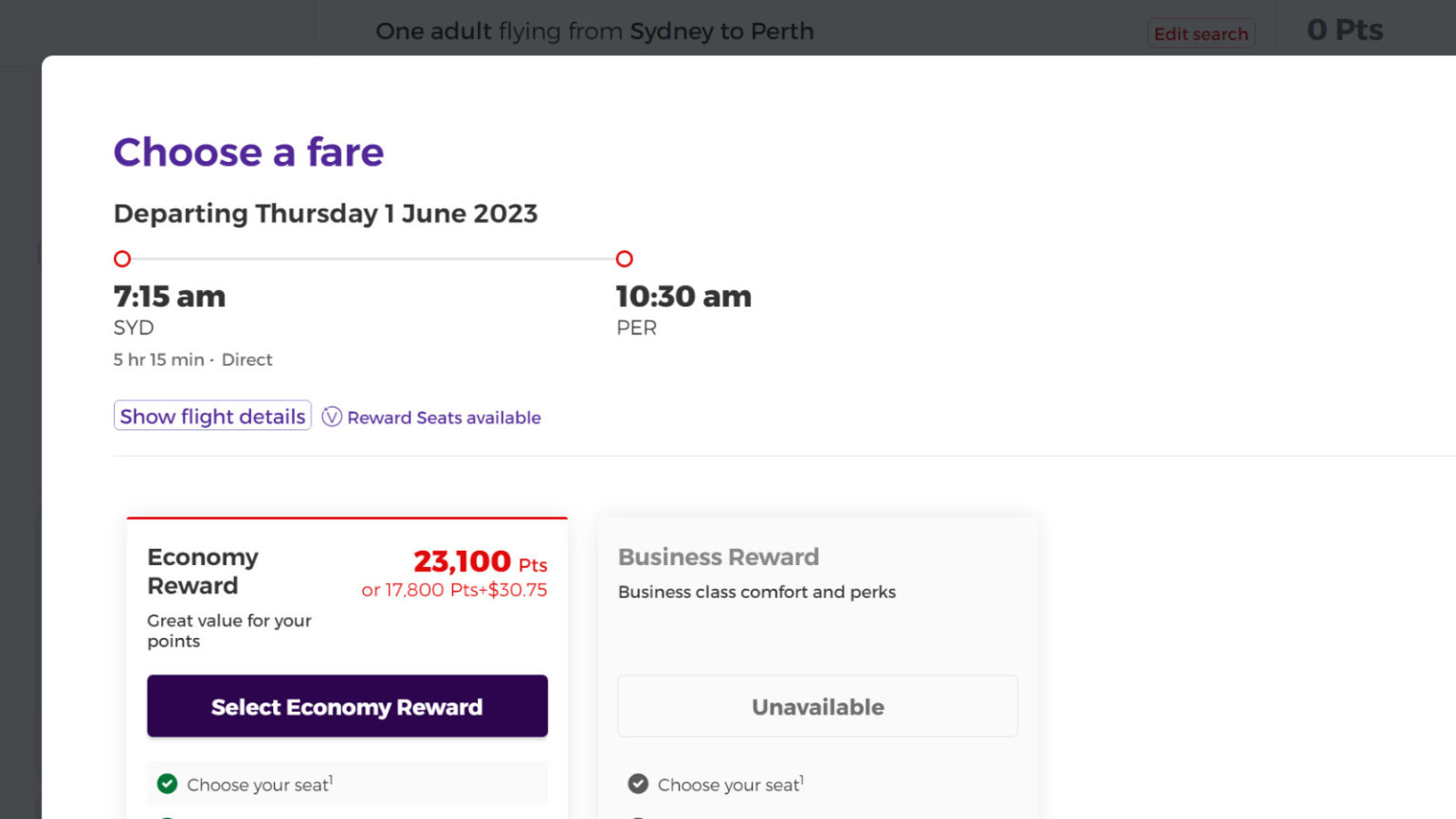This web page on an airline booking website allows users to select their fare options for a flight. The interface features a slightly darkened border highlighting a booking for one adult traveling from Sydney (SYD) to Perth (PER). Users have the option to edit their search or see that they have zero points.

Within the main section of the page, beneath the heading "Choose a Fare," details for the departure are provided: the flight is scheduled for Thursday, June 1, 2023. A visual timeline shows a circle connected by a line to another circle, indicating the direct flight's schedule starting at 7:15 a.m. from Sydney and arriving at 10:30 a.m. in Perth, with a total flight duration of 5 hours and 15 minutes.

A box labeled "Show Flight Details" is available for more information. Additionally, a circle with a "V" inside indicates that reward seats are available on this flight. Below this, two fare options are presented. 

The first option on the left, currently selected, is for an Economy Reward fare. It offers a choice between 23,100 points or a combination of 17,800 points plus $30.75, promising value for your points. There is a prominent purple button with white text that reads "Select Economy Reward," along with a green circle with white text that says "Choose your seat."

The second option on the right is for a Business Reward fare, which offers business class comfort and perks. However, this option is currently grayed out and unavailable. A gray circle with a white check within also indicates the option to choose your seat if it were available.